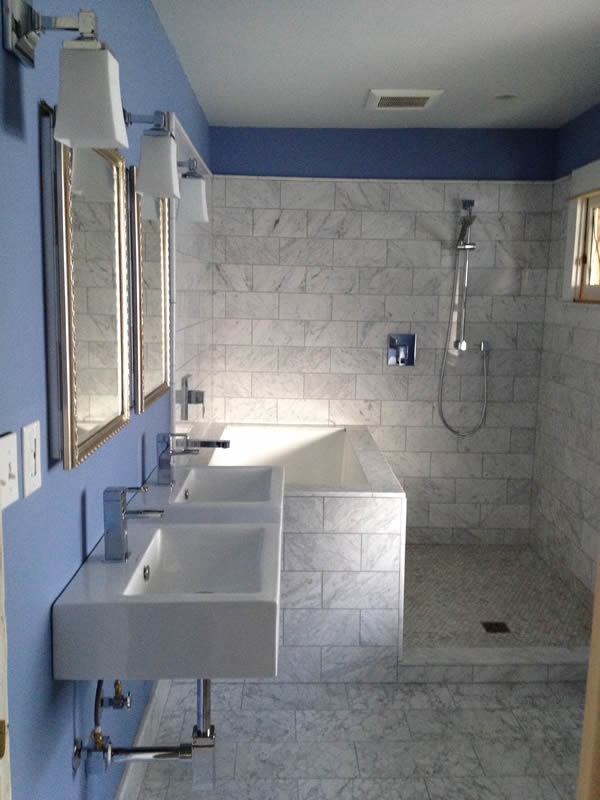This image shows a modern and stylish bathroom. The left wall is painted a pretty sky blue and features two large, rectangular mirrors with elegant gold frames. In front of the mirrors are two square, white porcelain sinks, each with a contemporary faucet designed to create a waterfall effect. Above the mirrors, there are three lights, adding ample illumination to the space. The floor is a mix of gray and white tiles, complementing the overall design. 

To the right of the sinks, there is an open shower stall with a silver, handheld shower head attached to the wall, allowing for flexible use. The walls in the shower area are covered in white brick tile, matching the tile that lines the bathtub situated immediately behind the sinks. A window on the right wall adds natural light to the room, enhancing its inviting atmosphere. The bathroom features a combination of blue painted walls and white brick tiles, creating a harmonious blend of colors and textures.